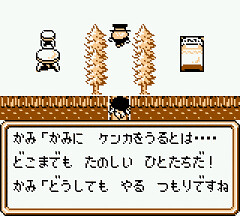This image, likely a screenshot from a video game, features low-resolution graphics with predominantly brown, white, and black colors. At the bottom of the image, there is a large white rectangular box containing black text in either Chinese or Japanese script, which is unreadable. The scene includes a few brown trees, and a character seems to be in mid-jump above these trees, located centrally in the image. To the left, there is an indistinct object that resembles a chair positioned near the middle of the screen. On the right side, there is a small box floating in mid-air. The ground is depicted as a brown surface with some yellow patterns. The overall aesthetic suggests it hails from an early-era video game.